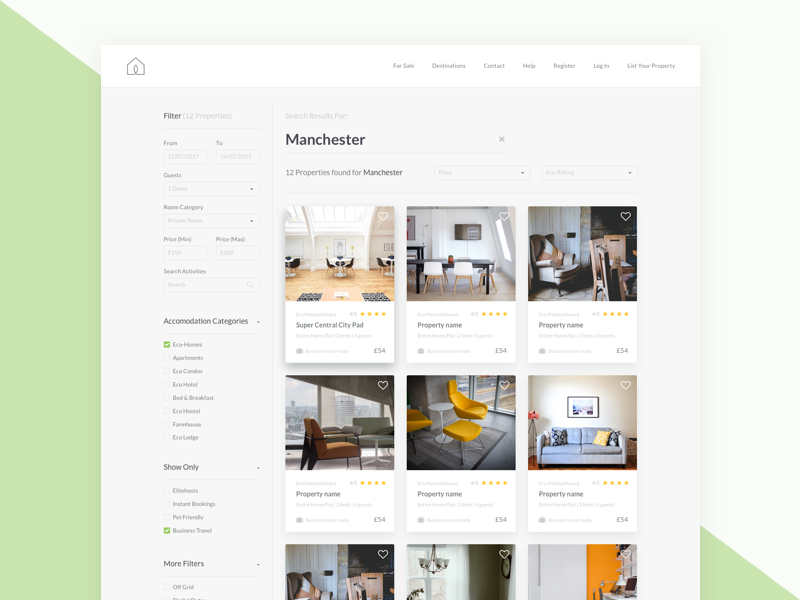The image depicts a user interface of a real estate rental website focused on properties in Manchester. The site displays a search result indicating "12 properties found for Manchester" and appears to have customizable filter options to refine the search results according to user preferences. The website design includes a distinctive color scheme with a lime green diagonal dividing it from a white background.

Prominent on the interface is a section labeled "Accommodation Categories," allowing users to categorize their search to better target their needs. There are nine property listings showcased, predominantly featuring interior images that suggest these properties are apartments or condos rather than standalone houses. Each listing includes user-generated ratings, providing feedback on the properties.

At the top of the page, navigation options include filters to view properties "For Sale," a contact section, a login portal for returning users, and a feature allowing property owners to list their rental spaces. The polished and user-friendly layout is complimented by a lime green and white color theme, enhancing the browsing experience.